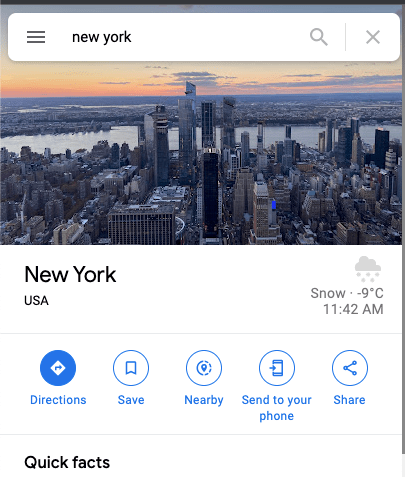In this mobile app-style image, which is vertically oriented, the upper left corner features a white text box containing three horizontal lines next to the word "New York" indicating the city. To the right of this is a search icon, followed by a close "X" on the far right. The central portion of the image showcases a stunning skyline view of New York City, taken from what is likely the Hudson River. The cityscape captures tall skyscrapers under a sky tinged with hues of orange and blue. Below the skyline image, text shows the current location and weather: "New York, USA" with conditions described as "Snow, -9 degrees Celsius," noted at "11:42 a.m." 

Further below, a series of interactive buttons are displayed for user convenience: "Directions," "Save," "Nearby," "Send to your phone," and "Share," with the "Directions" button highlighted in blue. Positioned in the lower-left corner, there is a bold, black-font area labeled "Quick Facts."